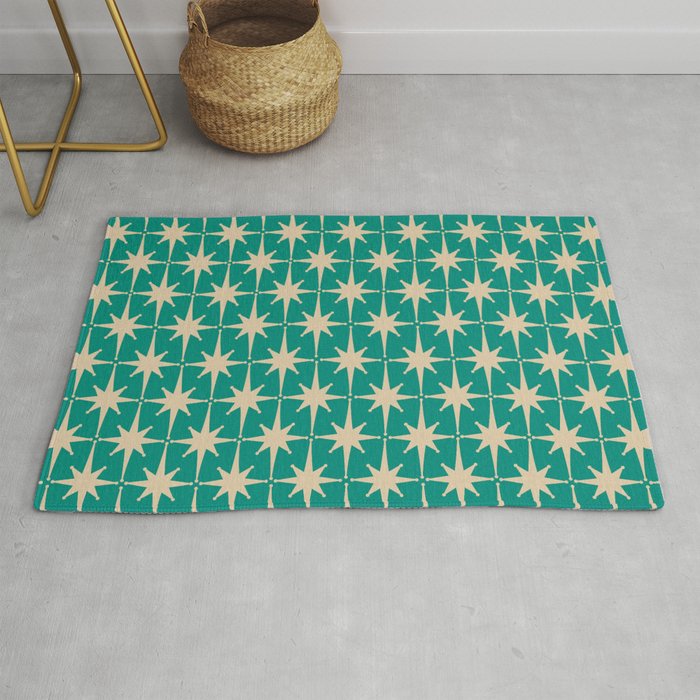This photograph captures an indoor scene with a squared composition, showcasing a centrally focused green floor mat adorned with numerous white starburst patterns intersecting at their tips. The mat, estimated to be rectangular around 3 feet by 2 feet, is placed on a light gray carpeted floor that features subtle white wavy accents. In the upper left corner of the image, part of a table or chair leg, shaped like a cross frame, can be seen. Adjacent to this, there is a woven cylindrical basket with handles, likely made of bamboo, positioned near the white-painted wall that forms the backdrop. The photo's setting suggests it could be a living room or an artist's studio, illuminated by artificial lighting, capturing the detailed textures and colors of the room.